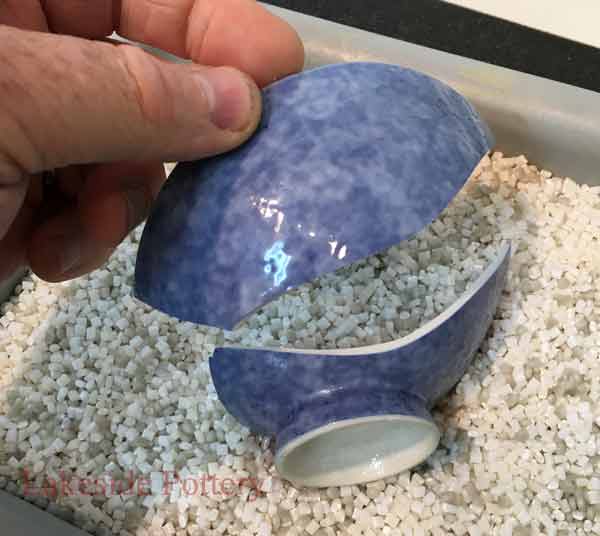In this image, a large hand, coming from the upper left corner, is holding a broken piece of what seems to be a ceramic vase. The piece in the man's hand displays a mix of light and dark blue hues. Below it, the lower half of the vase, including the spout or opening, rests on a bed of white and gray pellets. This section is primarily white on the inside. Both pieces of the vase exhibit a vivid blue color, with the piece in the hand showcasing a more intense blue, transitioning from light to dark shades. The entire scene is set inside a gray plastic or fiberglass container, adding a rugged contrast to the delicate shards. The purpose behind the setup is unclear, whether the man intends to repair the vase or simply display its broken state.